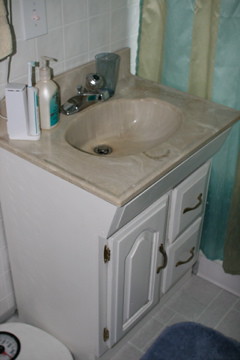This photograph captures a compact bathroom setting, presenting a single sink with minimal counter space. The countertop appears to mimic beige granite but is likely made of plastic. The bathroom walls are adorned with pristine white tiles featuring white grout. Below the sink, a white-painted cabinet with one door and two drawers offers some storage space. A white bathroom scale is positioned on the floor beside the cabinet. 

The countertop hosts a few essential items, including a white and green electric toothbrush in its holder, a pump bottle of hand soap, and a gray glass. Adjacent to this setup, a blue and yellow (possibly gold or beige) shower curtain is partially visible, indicative of the bathtub or shower area. A light switch is mounted on the wall above the counter, though no mirror is visible in the frame—possibly installed higher than what the photograph displays. 

Adding to the bathroom's subtle detailing, a beige towel hangs above the toothbrush, contributing to the room's functional decor. The flooring consists of white tiles that match the walls, with a blue rug laid out to offer a touch of comfort and color contrast to the otherwise neutral palette.